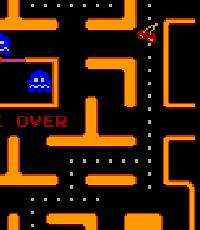This is a detailed screenshot of the classic Pac-Man video game, showcasing the lower right portion of the playing field. The maze is composed of bright orange barriers set against a black background, with white dots scattered throughout pathways—some of which have already been eaten by Pac-Man. In the upper right corner of the capture, two red cherries are visible on a path. Two ghosts are present: one partially visible in the upper left and the other in the center, both turned blue, indicating they can be eaten by Pac-Man. Below the central ghost is the digital orange word "OVER," signaling a game over scenario. This close-up view illustrates roughly 20% of the game screen, with tunnels extending off to the sides, leading to a larger maze structure.